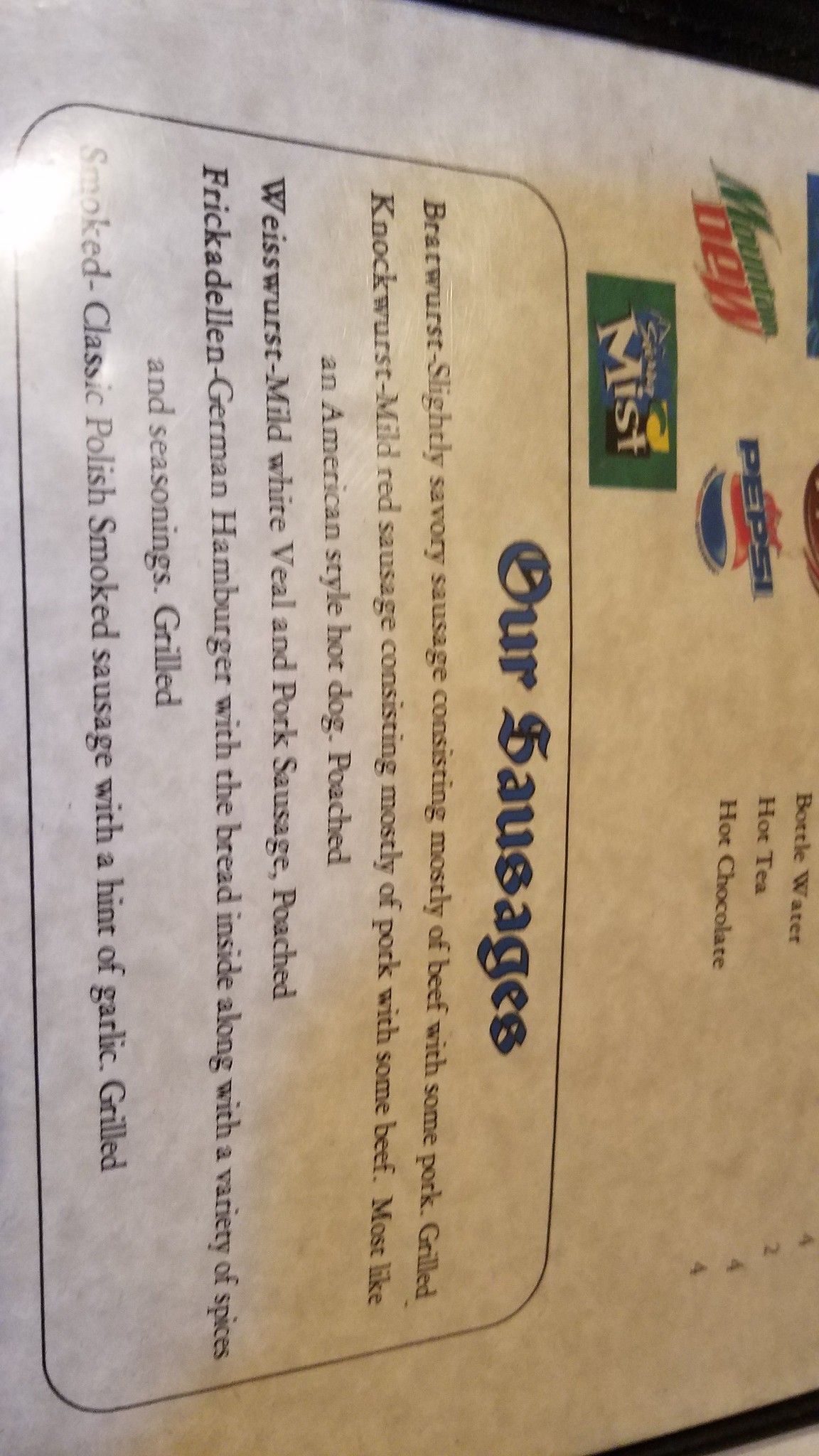This image captures the bottom portion of an open menu, framed by a black border on both the right and left sides. The upper left section of the page features a list of various beverages, including soft drinks like Mountain Dew, Pepsi, and Sierra Mist. In the upper right corner, additional drink options are listed, such as bottled water, hot tea, and hot chocolate. Dominating the bottom half of the page are detailed descriptions of specialty sausages the establishment offers. These include Bratwurst, a slightly savory sausage; Knackwurst, a mild red sausage made from pork and beef, poached; Weisswurst, a mild white sausage composed of veal and pork, poached; Frikadellen, described as a German hamburger; and a Smoked Classic, which is a Polish smoked sausage with a hint of garlic, grilled to perfection. This descriptive section provides a rich overview of the menu's offerings, adding to the visual appeal and culinary allure of the page.